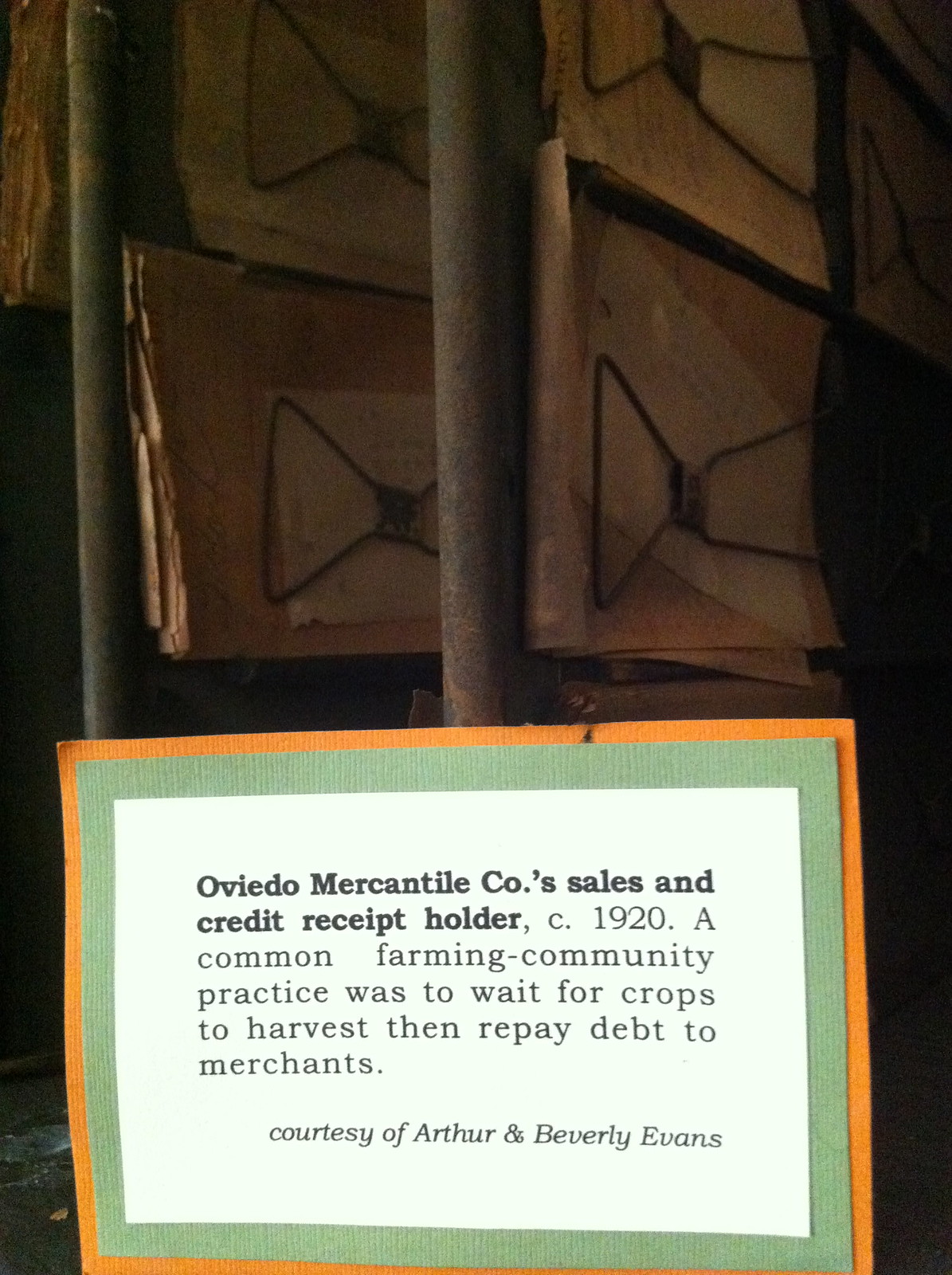The image is a full-color photograph showcasing a collection of artifacts prominently displayed against a backdrop. In the lower portion of the image, three horizontally rectangular pieces of fabric are arranged: an orange fabric at the bottom, overlaid by a green fabric, and topped with a white paper sign. The sign, bordered by the green and orange fabrics, contains black text that reads, “Oviedo Mercantile Company's Sales and Credit Receipt Holder, circa 1920. A common farming community practice was to wait for crops to harvest, then repay debt to merchants." The sign also notes that it is "Courtesy of Arthur and Beverly Evans." The sign appears affixed to a rusted, black iron bar, indicative of aged metal pillars, with additional bars and clips holding aged papers behind it. The backdrop comprises various brown elements, possibly old receipts or documents, further emphasizing the historical context of the farming community’s credit practices.